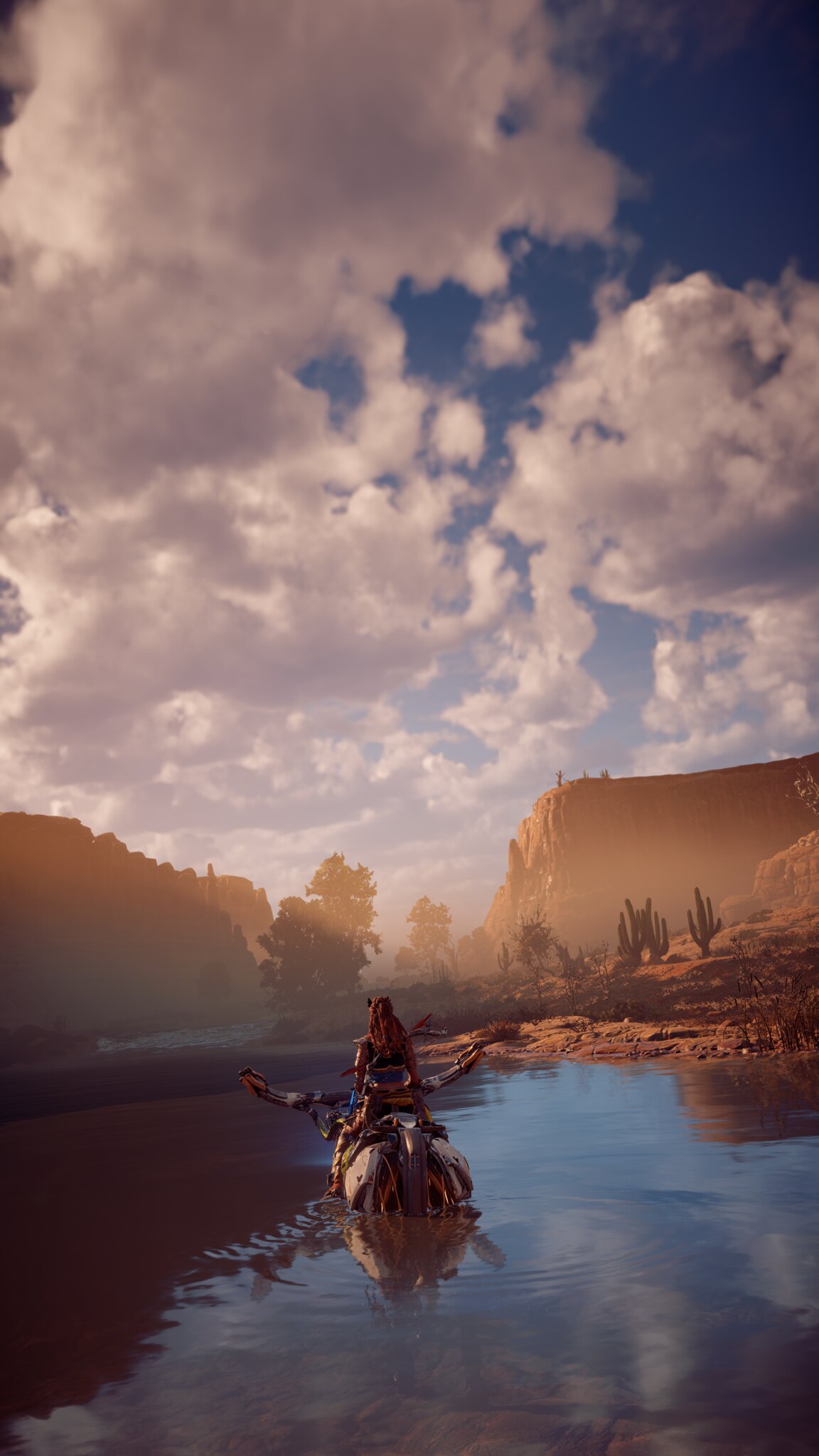This artwork depicts a serene and evocative scene centered around a solitary figure. Positioned at the heart of the image, the person, viewed from the back, is riding on an indistinct object. Their long, brown hair cascades down to their back, adding a subtle detail to their silhouette. Above them, a predominantly cloudy sky fills the upper part of the canvas, with scattered patches of blue peeking through, hinting at a calm and overcast day. Below, the figure and the object they ride are situated within a tranquil body of water, adding to the serene ambiance of the scene. The background is rich with natural elements, featuring a variety of greenery. On the left side, a group of trees contributes to the lush landscape. Centrally, a cactus stands out, adding a touch of the arid to an otherwise aqueous setting. To the right, in the distance, rolling hills and cliffs rise, providing depth and a sense of place, further anchoring the scene in a diverse natural environment.